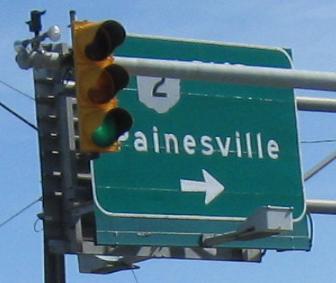This square color photograph captures a clear view of a highway sign against a light blue sky. The dark green sign, adorned with a thin white border, features white text that possibly reads "Paynesville," though the initial letter is obscured by a yellow traffic light. The illuminated green light, indicating 'go,' partially blocks the first letter. Adjacent to the visible sign, a secondary sign is conjoined by a central steel structure. An arrow pointing to the right suggests the direction towards Route 2, which is denoted by a black numeral "2" on the sign. The entire scene is framed by silver metallic supports, adding to the utilitarian aesthetics of the highway infrastructure.